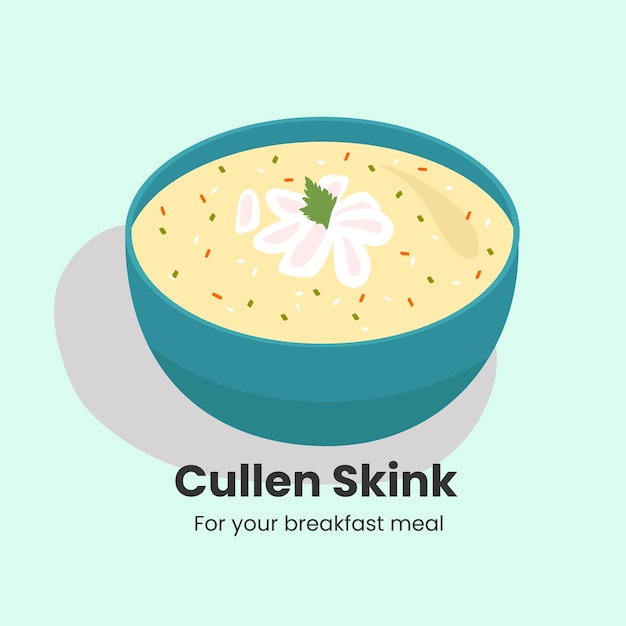The image portrays a cartoonish illustration of a breakfast meal called "Cullen's Skink." Set against a seafoam green background, a blue bowl holds a light yellowish-beige soup. The soup is dotted with green and reddish-orange bits, giving it a colorful appearance. Central to the composition is a decorative design, likely representing a flower with a parsley leaf at its center. The bowl casts a subtle shadow against the background, adding depth to the simple yet visually appealing scene. The accompanying text, using a combination of black, green, grey, and butter colors, reads "Cullen's Skink for your breakfast meal."